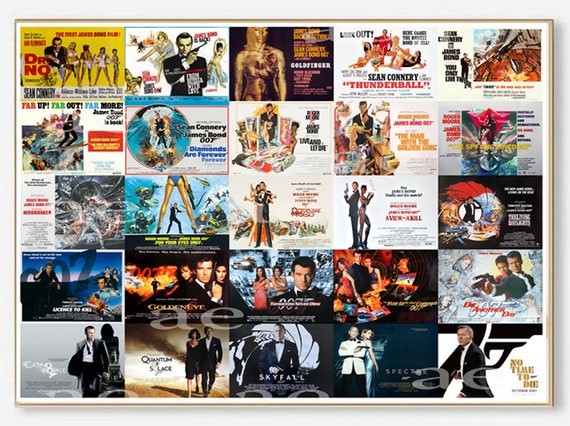The image is a meticulously arranged collage featuring 25 distinct James Bond movie posters, organized in a 5-by-5 grid. Each square, representing a different film, highlights the iconic franchise's evolution, starting with "Dr. No" in the top left corner, which showcases James Bond alongside four women with the title boldly written in red. The collection spans decades, capturing classics like "Goldfinger," "Moonraker," "Thunderball," and "The Spy Who Loved Me," and extends to more recent additions such as "Skyfall" and "No Time to Die." Across the collage, the faces of various Bonds, with a notable concentration on Sean Connery and ending with Daniel Craig, paint a historical timeline of the series. In the midst of this vibrant assembly, the lettering "A&E" is prominently displayed. Each movie poster is distinctly colored, creating a visually striking homage to the legendary 007 series.